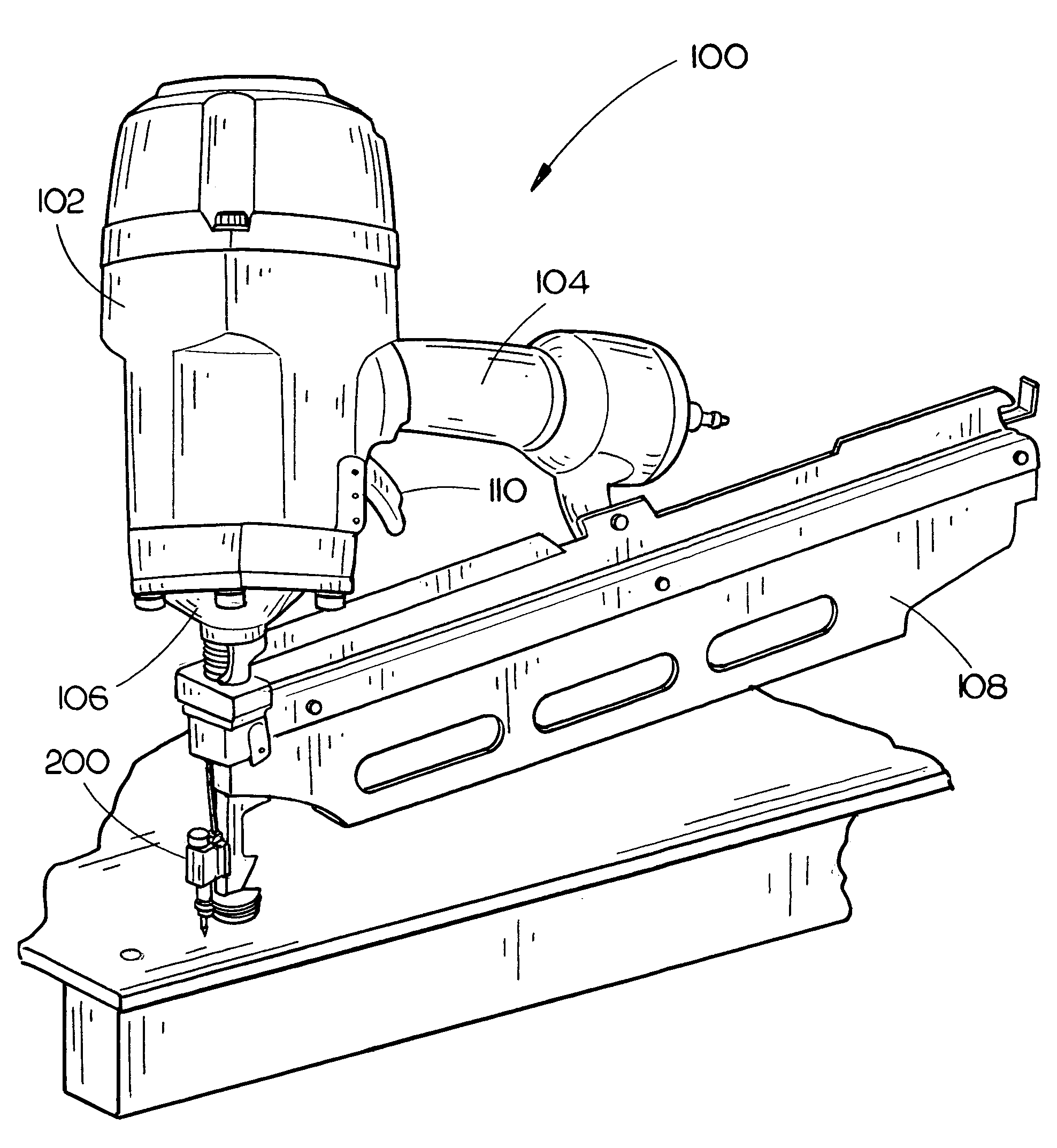This is a detailed black-and-white sketched diagram of a pneumatic nailer, depicted on a simple white background. The tool is oriented facing downward, with its handle extending to the right and the back end positioned at the top of the image. Various components of the nailer are labeled with numbers such as 100, 104, 110, 102, 106, 200, and 108, though the legend for these numbers is not visible. The nailer features a long canister-like body and a handle that extends approximately two inches before widening into a larger bulbous end, with a trigger in front of the handle. The diagram highlights several key parts of the tool, including the air hose connection, nail feed area, and the head that drives the nails. A logo is present on the nailer, but it is unreadable, leaving the brand unidentified. The nailer is depicted in the act of driving into a flat piece of wood, which shows sawed edges on its backside and right side.